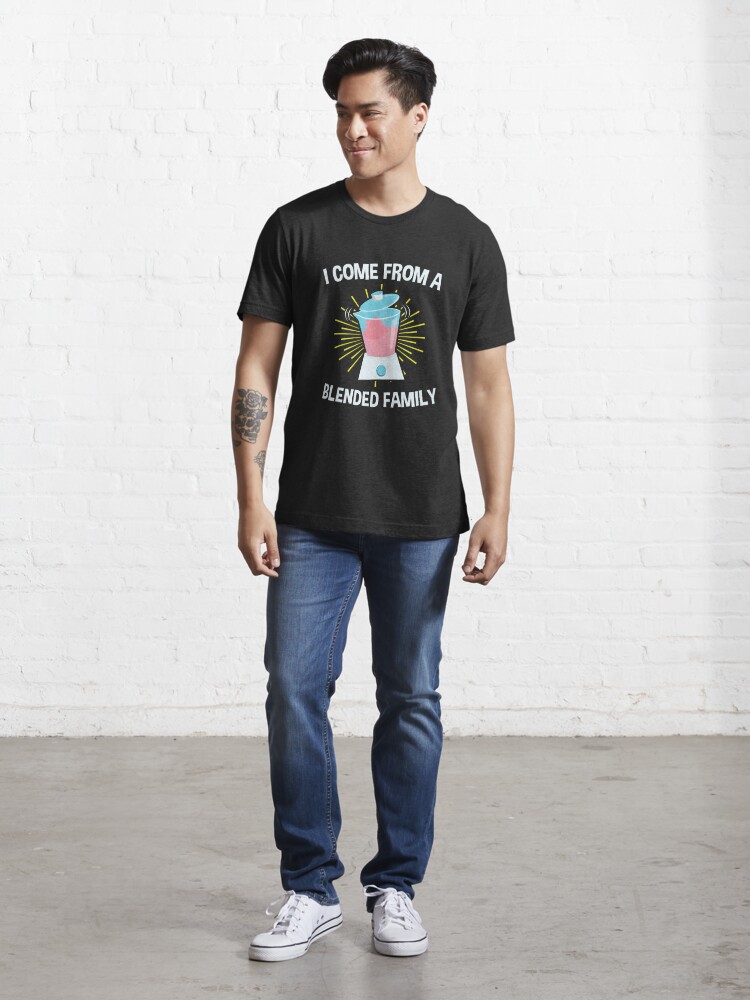In this detailed color photograph, we see a young man standing in a minimalist concrete room with gray cement flooring and a white brick-styled wall. He has black hair and a smirk on his clean-shaven face. His head is turned to his right, looking off into the distance.

He is dressed casually in blue jeans and white Converse sneakers. His black t-shirt prominently displays a playful graphic reading "I come from a blended family," featuring an image of a green blender overflowing with pink contents. The blender's top is depicted coming off, with yellow spikes radiating from the blend. His right forearm is adorned with tattoos, including a skull with flowers and another design that looks like a dog or a seal, while his left arm is free of any tattoos.

The tall, lean man appears to be posing, possibly modeling, as he exudes a relaxed, confident demeanor amidst the stark, industrial setting.